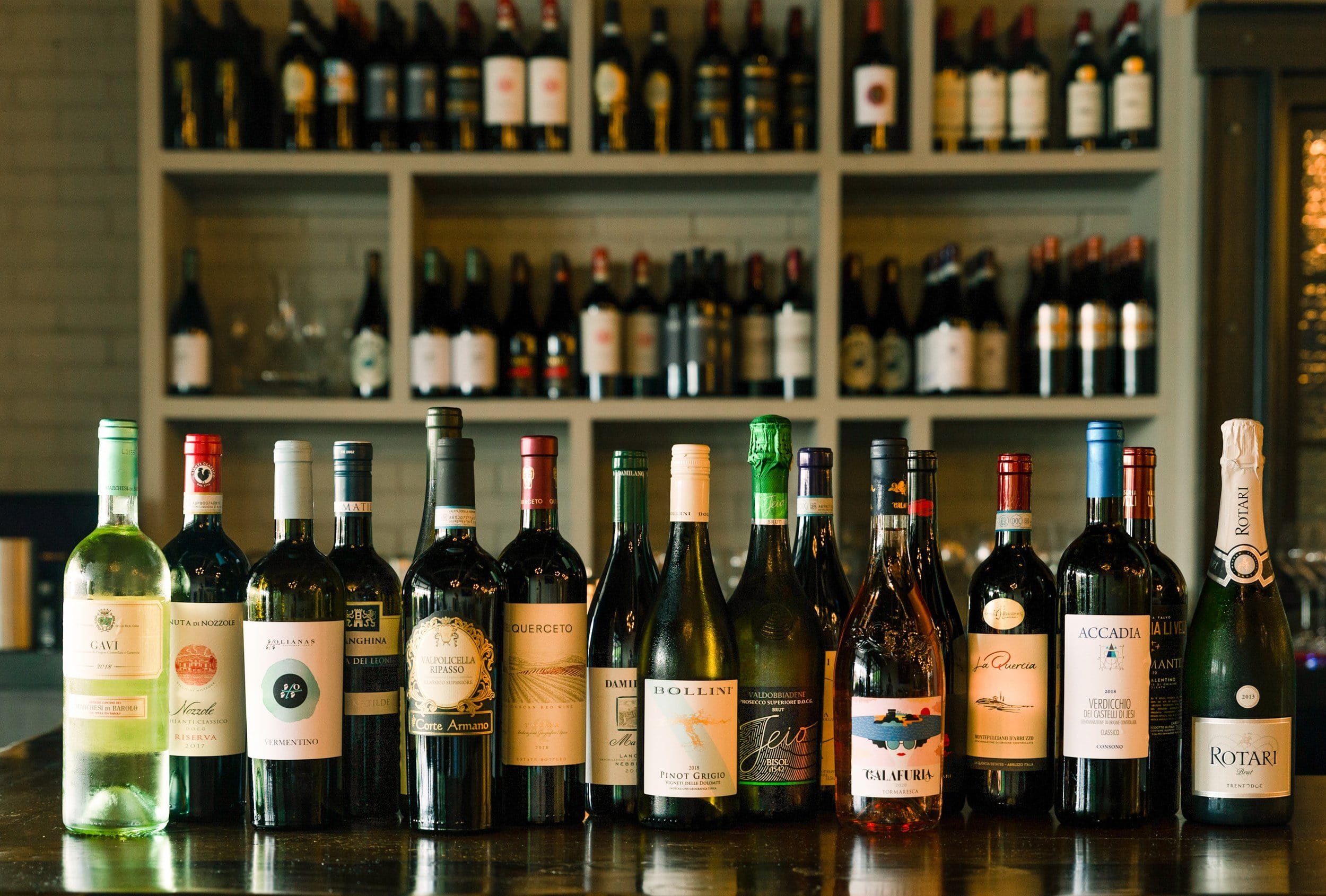The photograph captures a vibrant display of multiple varieties of wine bottles meticulously arranged on a glossy, reflective brown counter at what appears to be a wine store, restaurant, or tasting venue. The composition features an array of wine bottles in the forefront, each distinct in shape and label: the leftmost being a clear bottle with green liquid, adorned with a white label and green cap, followed by a green bottle with a red cap and white label, another green bottle with a blue cap and white label, a black bottle with a white and green label paired with a black cap, and finally, another black bottle showcasing an ornate white label. In the background, a gray painted brick wall supports shelves brimming with additional wine bottles, contributing to the overall ambiance. Although slightly blurred, the backdrop highlights the establishment's extensive wine collection, with tantalizing glimpses suggesting a broader array of spirits or perhaps other gourmet items, carrying the potential of being mistaken for olive oil bottles. The surroundings hint at a well-furnished locale, with notable elements like a door with brown borders and a wall featuring brick patterns, perhaps housing an oven, adding to the venue's cozy, inviting atmosphere.